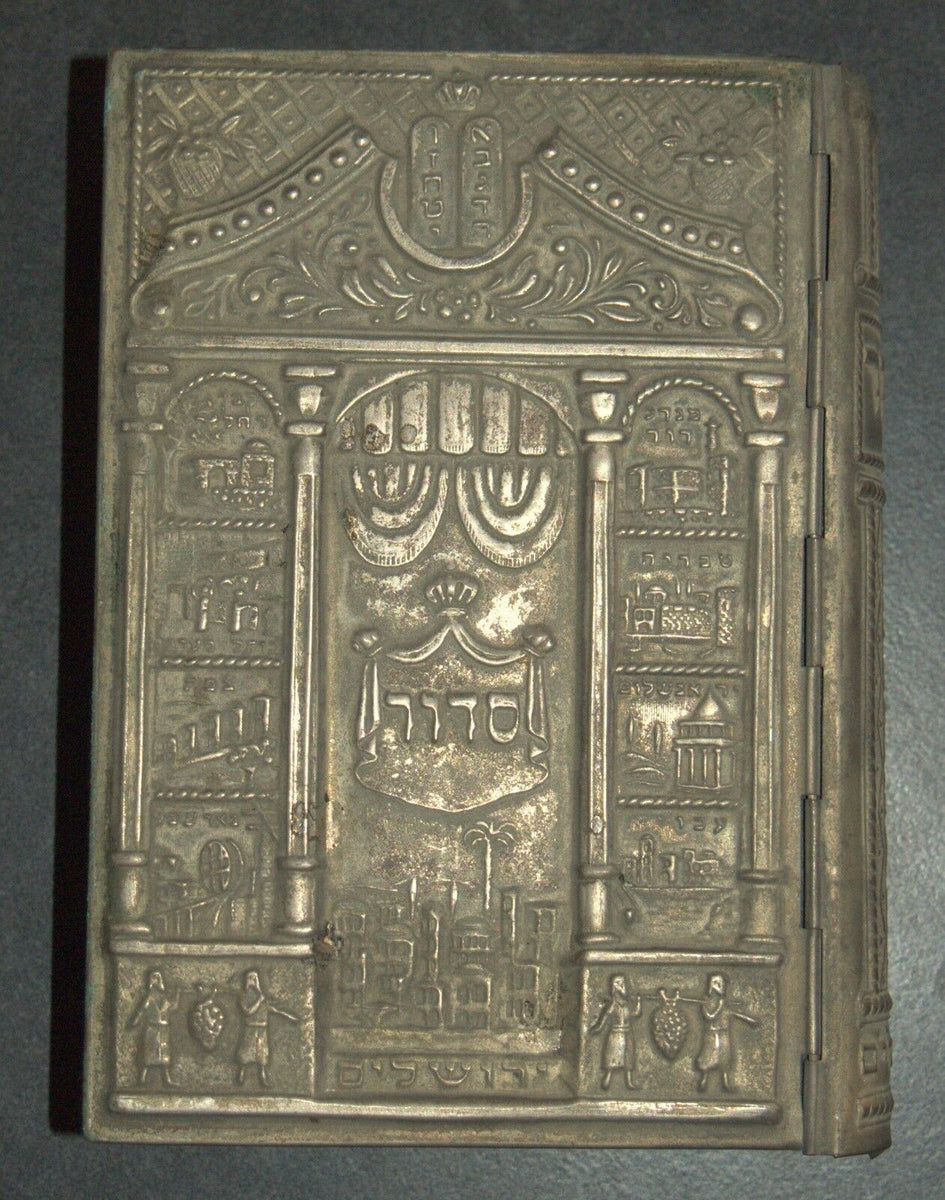The color photograph in portrait orientation showcases a vintage Siddur Hebrew Prayer Book, prominently detailed and adorned. The cover, made of a dark bronze, exhibits shiny highlights that enhance its intricate design. At the top, the book features a decorated pediment-like arc, housing two central plaques inscribed with ancient Hebrew writing. Below this are four vertical columns, framing a central opening that displays a carved cityscape at the bottom, over which drawn-back curtains hang, also marked with Hebrew characters. The bottom section of the book's cover vividly portrays two men, each holding a stick over their shoulders, from which a significant item, possibly an animal or a large bundle, is suspended. Additional carvings adorn the entire surface, each small square etched with scenes that narrate stories, all rendered in a photographic realism representationalism style. The left side of the book is equipped with hinge-like features, complementing the hard, metal-bound, and heavily carved exterior that collectively tell the story and significance of this ancient artifact.